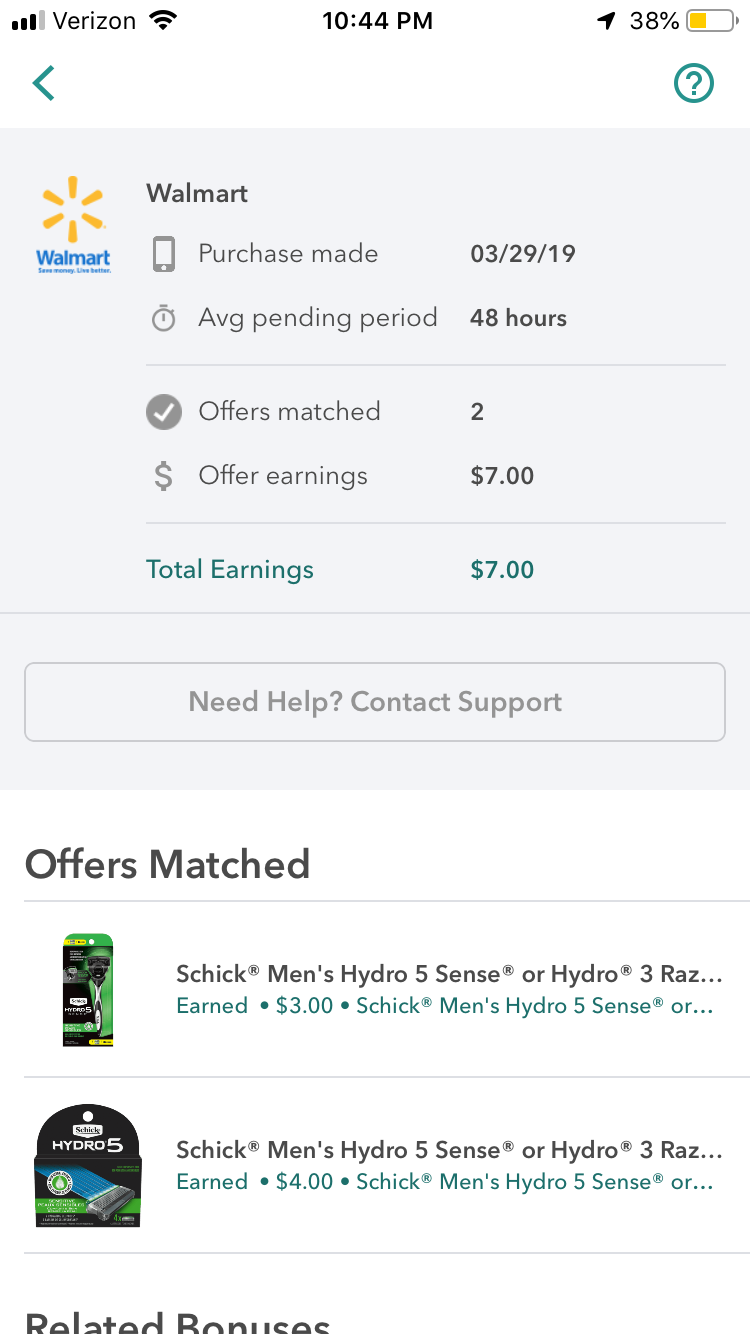In the upper left corner of the image, the cell phone company is indicated as Verizon, with the time displayed as 10:44 p.m. and the battery level at 38%. Below this is an order confirmation from walmart.com, featuring a series of short yellow lines forming a circle. Beneath these lines, the word "Walmart" appears in blue text.

The main portion of the image showcases a cell phone, accompanied by purchase details. The purchase was made on 3-29-2019, indicated next to a clock icon. The average pending period is noted to be 48 hours, marked by a check mark inside a circle. It also states that two offers have been matched, with "Offer Earnings" totaling $7, displayed next to a dollar sign. In green text, "Total Earnings" also shows $7.

A large rectangular section below provides an option labeled "Need Help? Contact Support," which is clickable. Further down, a section labeled "Offers Matched" features an image of a razor inside a box. Beside this image, it reads "Schick Men's Hydro 5," with earnings noted as $3. Another box below this details another offer for "Schick Men's Hydro 5," with $4 earned.